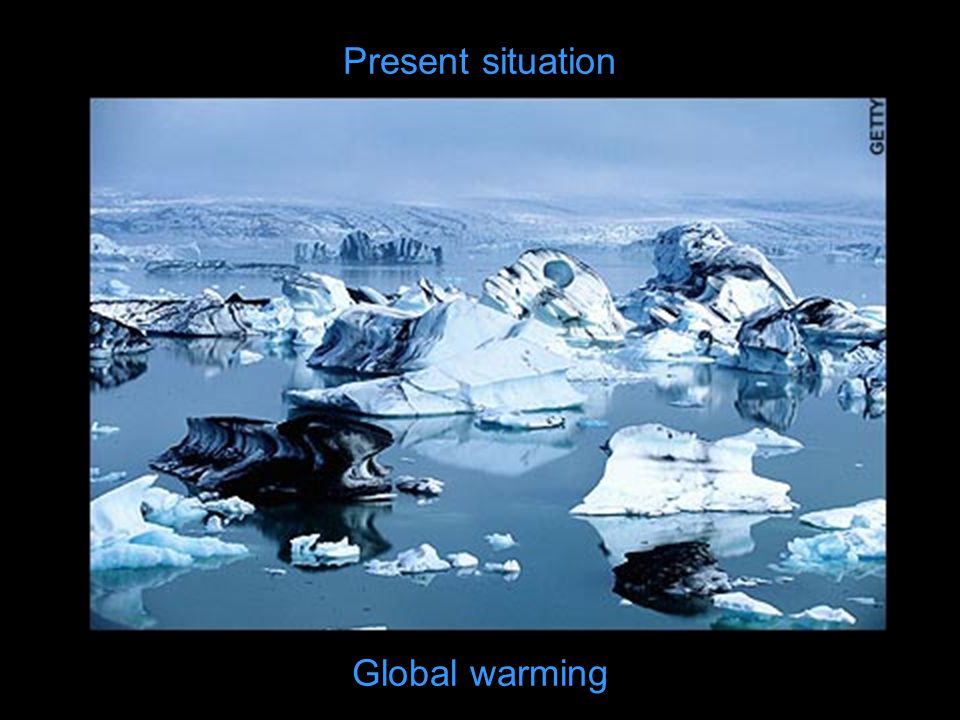This PowerPoint slide features a striking photograph set against a black background, depicting a scene from either the Arctic or Antarctic regions. Dominating the middle of the slide is an image of a sea filled with numerous icebergs, some of which appear darkened and partially melted, contributing to an ominous atmosphere. In the distance, muted tones of blue, black, and white reveal snow-covered hillsides or tundra. Above the photograph, in blue text, the slide is titled "Present Situation," while the same blue text at the bottom reads "Global Warming." The photograph is credited to Getty, noted in all caps in the top right corner of the image. This descriptive slide evidently forms part of a presentation addressing the impacts of global warming on polar landscapes.